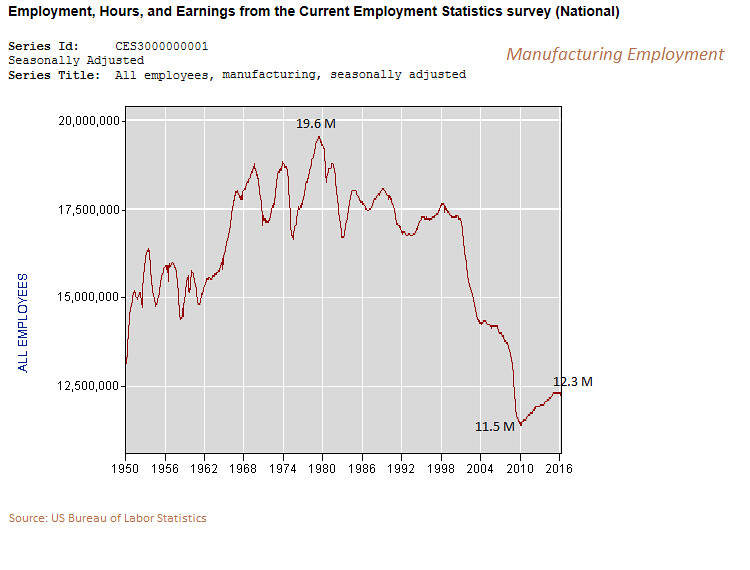The image displays a detailed statistical graph on manufacturing employment, titled "Employment, Hours, and Earnings from the Current Employment Statistics Survey National." Under the title, there are specific details, including a Series ID and the notation "seasonally adjusted". In the upper right corner, the label "Manufacturing Employment" is visible. The vertical axis of the graph tracks the number of employees, with data points highlighted in a red line, while the horizontal axis spans from 1950 to 2016. The peak manufacturing employment is noted at 19.6 million employees in 1980, while the lowest point is 11.5 million in 2010. By 2016, employment figures slightly increased to 12.3 million. The graph also indicates that the data is provided by the U.S. Bureau of Labor Statistics.